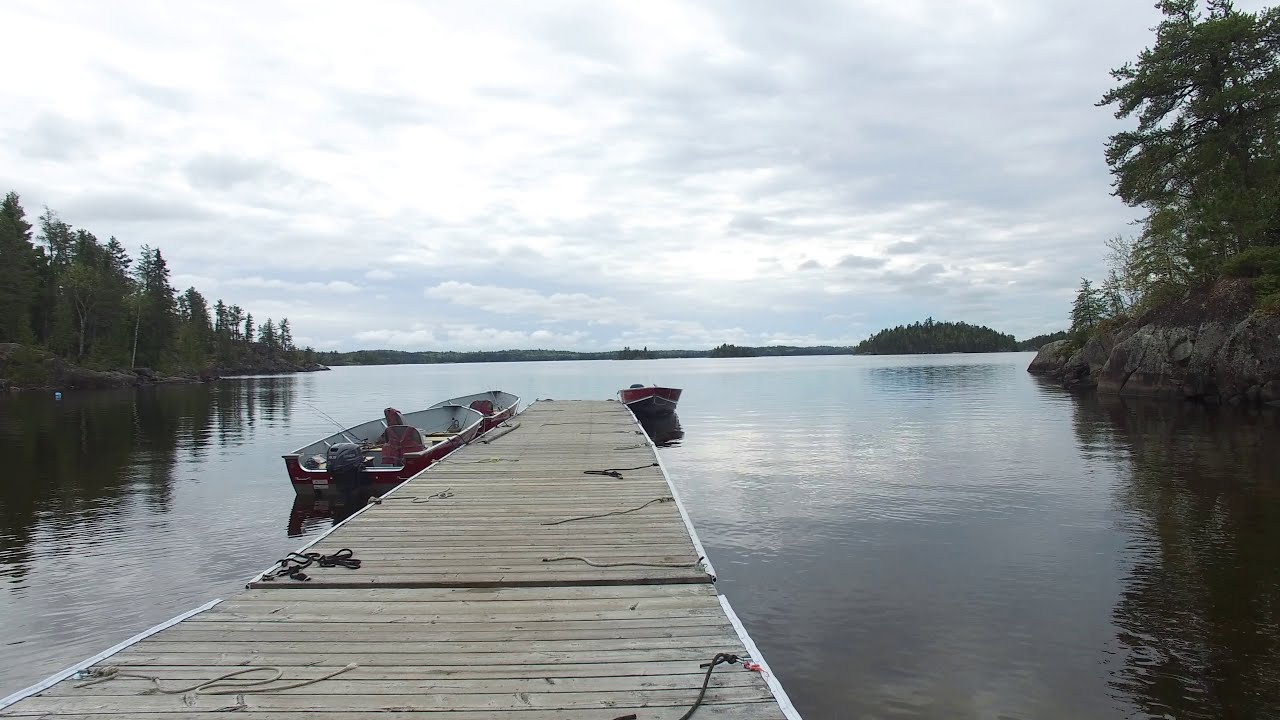The photograph captures a tranquil lake scene featuring a narrow, wooden dock extending from the foreground into the distance, disappearing into the calm, clear water. The dock's horizontal wooden boards create a rustic path leading to the lake's horizon. Scattered about the dock are ropes and three small outboard motor boats. Closer to the viewer, on the left side of the dock, a boat is tied up with a man sitting in it, possibly holding or resting by a fishing pole. Further out, two empty boats are moored at the end of the dock; one on the left, identifiable by its red chair and fishing equipment, and another boat that is partially visible on the right. Surrounding the lake on both sides are dense woods with tall trees, while the distant shoreline also appears lush with similar foliage. The sky above is overcast, filled with varying shades of white and gray clouds, contributing to the serene and still atmosphere of the scene.